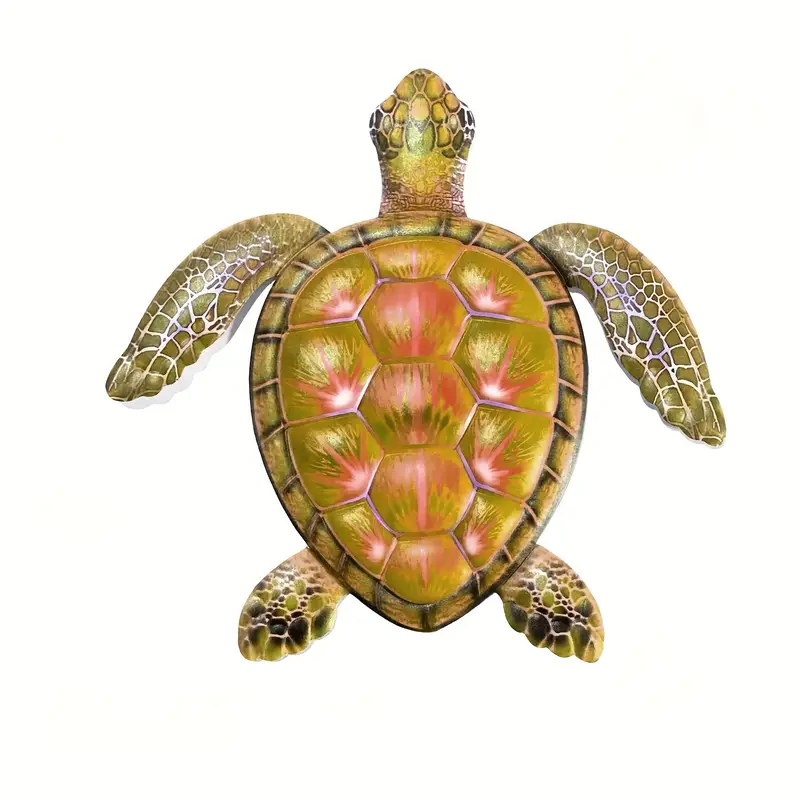This detailed image depicts a seemingly artificial sea turtle, possibly inflatable or a toy, rendered from a top-down perspective against a plain white background. The turtle’s shell, shaped like a teardrop with an oval top and pointy tail, is the focal point, showcasing a complex pattern with numerous sections. The outer edge of the shell is adorned with grooved lines in shades of brown interspersed with tan lines, which accentuates the intricate bumpy hexagonal shapes within, each featuring brown spikes resembling tiny explosions of light. The colors within the shell range from various greens and browns to tinges of yellow, pink, and white, adding a vibrant, almost dynamic appearance.

The turtle's fin-like front arms extend from the upper left and right, displaying an olive green hue interwoven with small white segments that create a veined look. Similarly, the back legs, positioned at the lower part of the image, are stubbier and showcase a green color with speckled dark brown and black highlights towards the bottom. The turtle's head, facing upwards as if swimming, has a green outline with sections shaded in olive and brown tones, highlighted with black near the eyes, which are positioned on either side. The neck transitions from primarily brown near the body to green closer to the head, merging the overall coloration harmoniously.